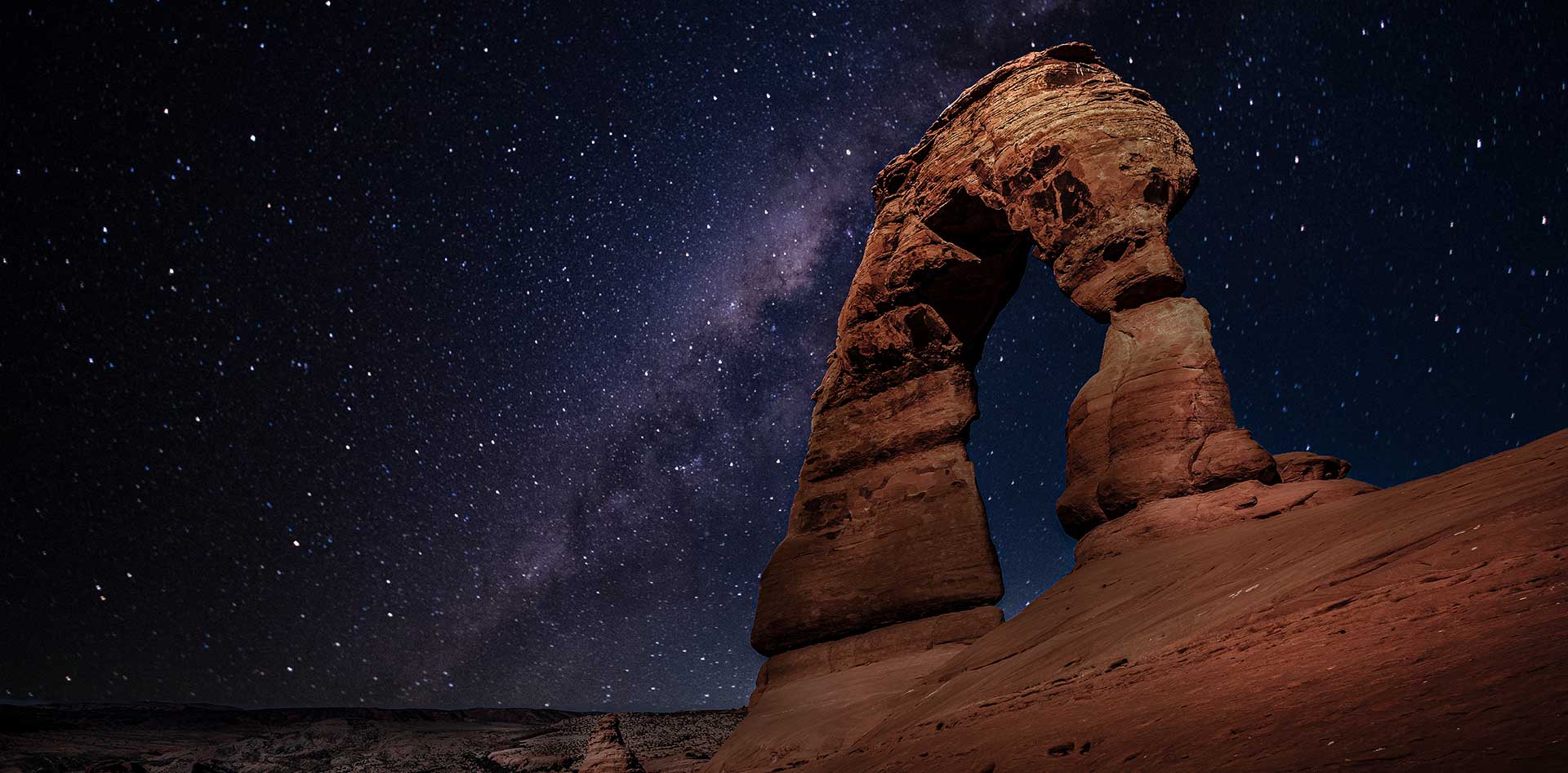The image is a striking depiction of a natural stone arch in a desert setting, captured at night. This impressive formation, resembling a lowercase "n" or a hollow doorway, stands tall on a rocky surface that stretches into the bottom right of the frame. The arch, weathered and eroded into its distinctive shape, showcases the intricate textures and earthy hues of brown, beige, and reddish tones. Behind this imposing structure, the night sky unfolds in a mesmerizing display. A vast expanse of black and blue is speckled with countless stars, and the magnificent Milky Way galaxy stretches across the center of the scene, adding to the enchanting nocturnal atmosphere. The image is exceptionally clear, providing a detailed view of the rocky landscape and the star-studded sky. Though it appears bright in certain sections, suggesting it might be a composite photograph or an artfully illuminated and manipulated image, the overall setting is unequivocally under the soft, natural glow of the night.